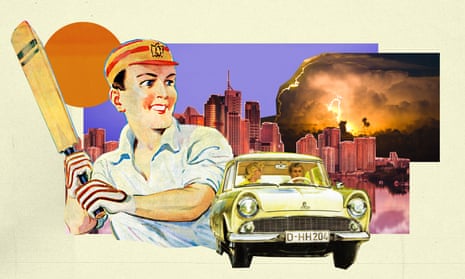In this detailed 1950s-style collage image, the composition features an array of elements superimposed to create a layered, nostalgic scene. The artwork is set against an off-white, eggshell border that frames a central field of muted purple. A skyline of skyscrapers stretches across the midsection, adding depth to the image. On the left side, a boy dressed in a blue polo shirt, orange-red striped gloves, and a matching hat holds what appears to be a cricket bat or perhaps a uniquely shaped object resembling a "crocodile bat." He stands poised as if about to swing. 

Adjacent to the skyline, extending to the top right corner, a dramatic scene takes place—cloud formations suggestive of a thunderstorm or possibly a more ominous event like a volcanic eruption or nuclear explosion, with lightning or plumes adding a sense of tension. 

At the bottom center, there's a vivid depiction of a vintage yellow car from the 1950s era, with a man in the driver’s seat and a woman beside him, engaged in conversation. Together, these elements create a complex, evocative image that blends mid-century Americana with surreal, collage-like visuals.